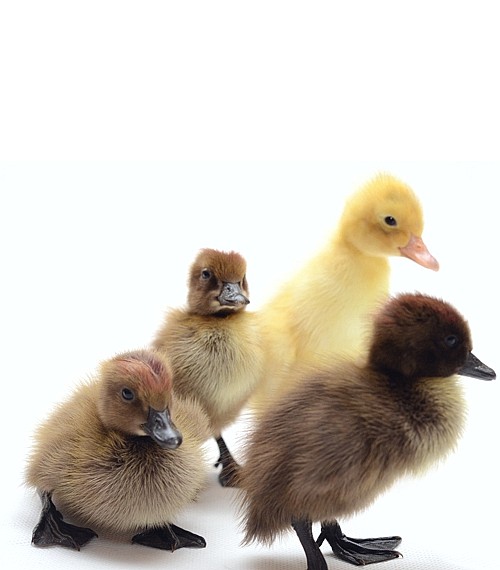In the image, there are four young, fluffy ducklings set against a light blue background with a white surface beneath them. The lighting from the upper left casts soft shadows to the bottom right, highlighting their youthful fluffiness. 

Starting from the left, two ducklings face more towards the camera; they both have light brown fur, dark brown beaks, and black feet. On the right side, one duckling at the bottom has a darker brown coat with black feet and a black beak. Behind it stands a taller duckling with bright yellow fur and a pinkish beak. All four ducklings appear very young, with their downy feathers contributing to their adorable and fluffy appearance.